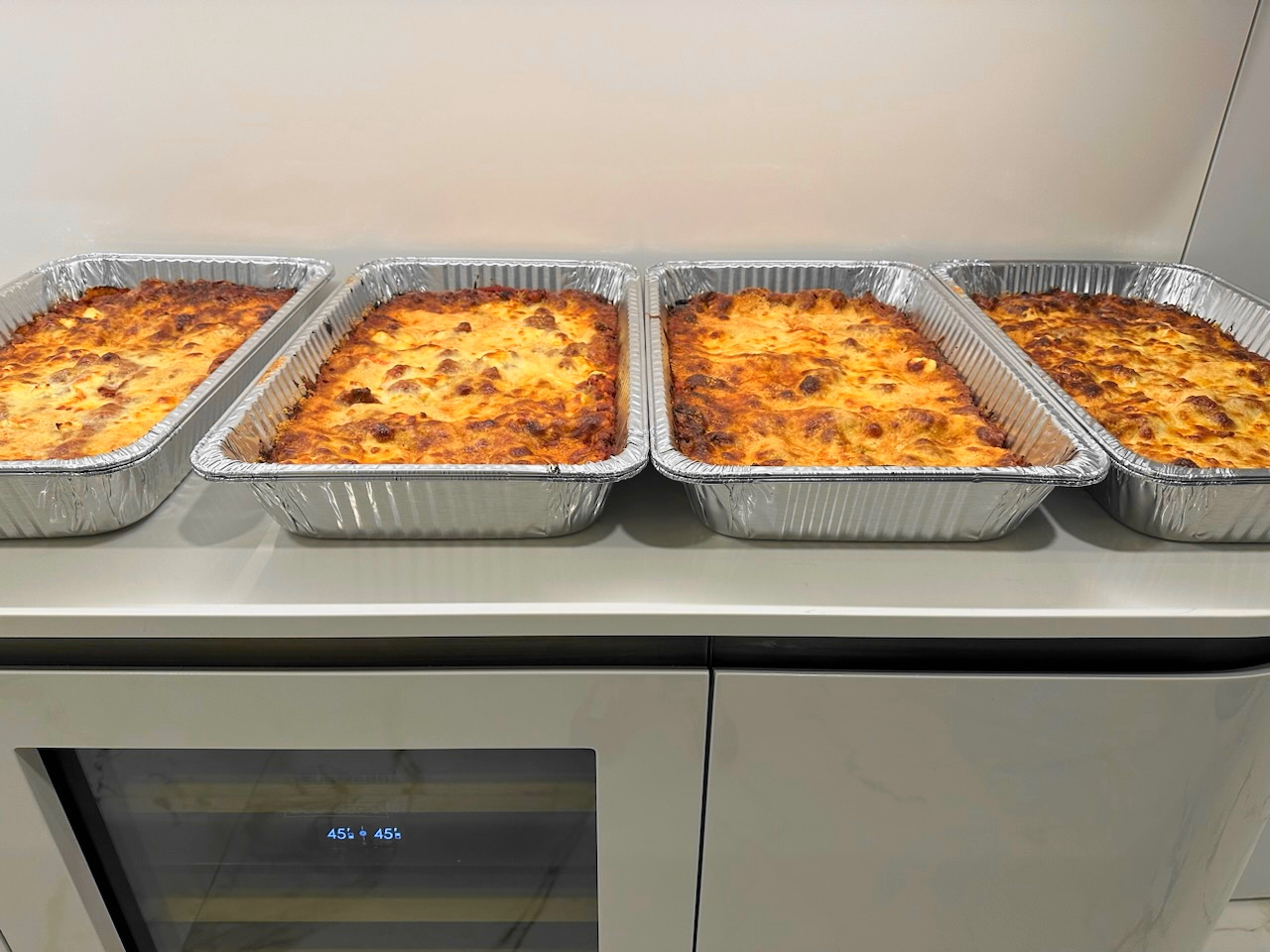This color photograph captures four large aluminum foil sheet trays, each filled with what appears to be a baked lasagna. The casseroles have a distinct yellowish-golden-brown, broiled cheese top, with edges that are slightly bubbled over and browned to a rich, appetizing color. The trays, which may be doubled for extra strength, are positioned on a metallic gray countertop. Below this surface, there is an appliance that could be either an oven, a heating tray, or a wine fridge. This appliance features a glass front with a digital display indicating "45" with a symbol in between, suggesting temperature control. The surrounding area includes a black strip above what might be a cupboard on the bottom right, and the white backdrop of a wall. The photo clearly illustrates the well-cooked, enticing nature of the lasagna, with melted, bubbling cheese that looks very appetizing.